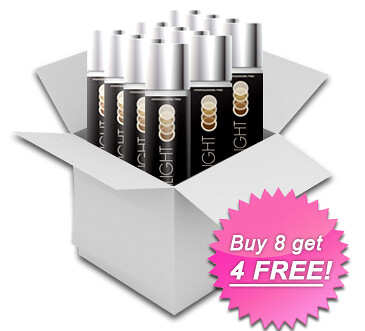This advertisement, likely for hair coloring products, showcases a detailed and visually appealing design. At the center is a white, three-dimensional box with open flaps, revealing a neatly arranged collection of 15 tall black cans, each topped with a silver cap. Each of these cans prominently displays the word "LIGHT" in white text and features small circles indicating various shades of brown, suggesting a range of hair color options. The box is positioned at an angle, giving it a dynamic, diamond-like perspective.

On the right side of the image, a striking pink circle with spiked borders commands attention. Inside this circle, white text emphatically announces a special offer: "Buy 8, Get 4 Free!" The words "4" and "Free!" are underlined and presented in a larger font for emphasis. The overall aesthetic gives the impression of a meticulously photoshopped or digitally drawn promotional material, possibly for makeup, lotion, or more likely, hair coloring products, given the visible details and the nuanced shades of brown displayed on each can. The vibrant offer and neatly packed products suggest a high-quality and appealing deal designed to attract consumers.